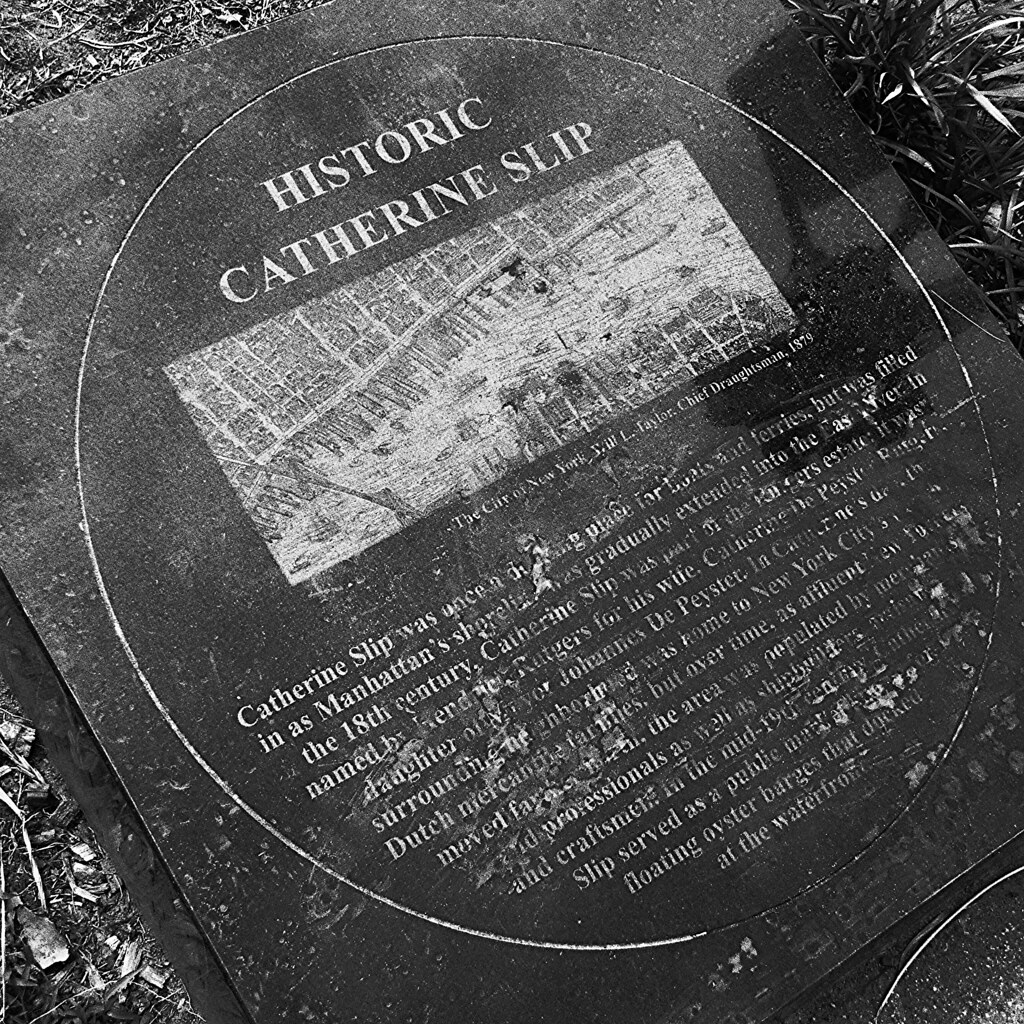The image is a close-up, black and white photograph of a historical plaque embedded in the ground. The plaque is a square stone with a circle inscribed in white at the center. At the top of the circle, it prominently reads "Historic Catherine Slip." Below this, there is a somewhat indistinct picture, possibly an old map of New York City. The text beneath the image is partially eroded and challenging to decipher but includes a reference to "the city of New York" and a narrative about Catherine Slip. The inscription suggests that Catherine Slip was an important location, initially a landing or pier, which was later filled in as Manhattan's shoreline extended.